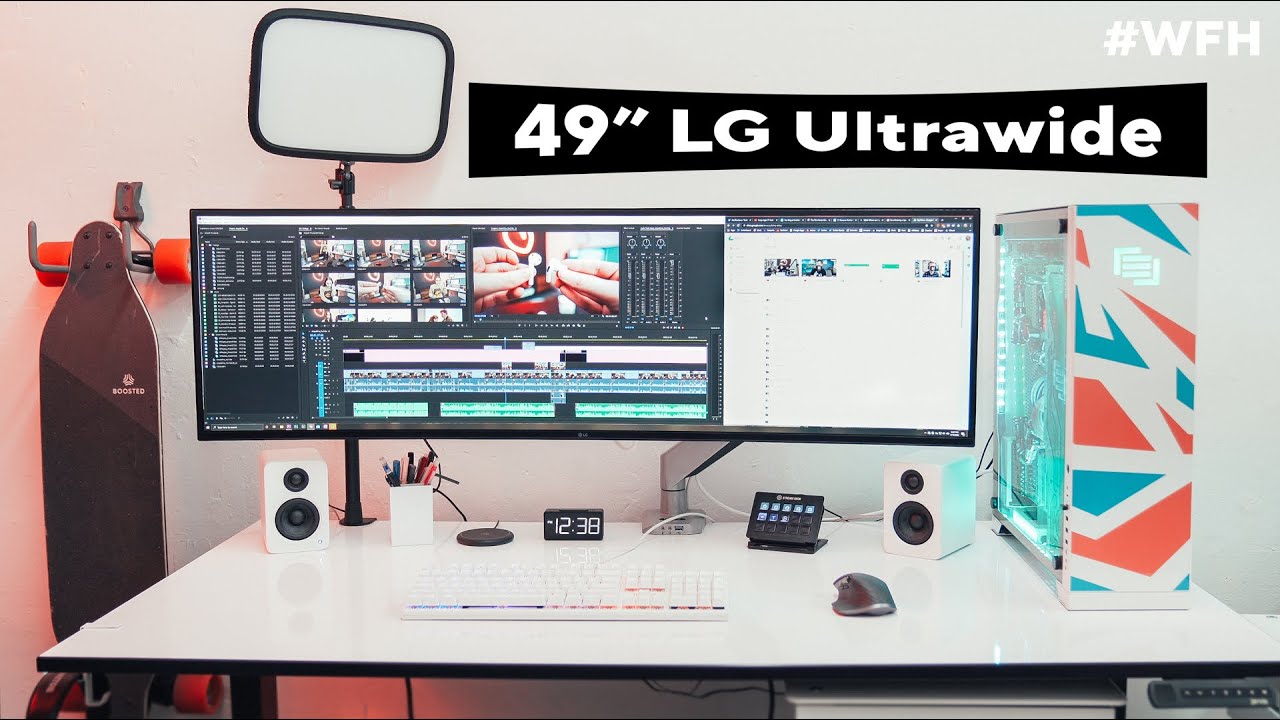The image showcases a modern PC setup on a spacious, flat, white desk. Dominating the scene is a 49-inch LG UltraWide curved monitor, prominently labelled with white text at the top. Above the monitor is a square light fixture, similar to a ring light but with a square design. Flanking the monitor are various desk accessories: a white speaker and cup filled with pencils on the left, along with a mirror attached to point towards the user, and another white speaker, a black mouse, a white keyboard, a stream deck with various buttons, and a small black alarm clock on the right. Positioned on the far right of the desk is a visually striking PC encased in a clear, blue, white, and red case, illuminated with green backlight. Completing the scene, a skateboard hangs on the white wall to the left of the desk, adding a touch of personal flair. In the top right corner of the wall, the hashtag "WFH" is displayed, underscoring the work-from-home setting.